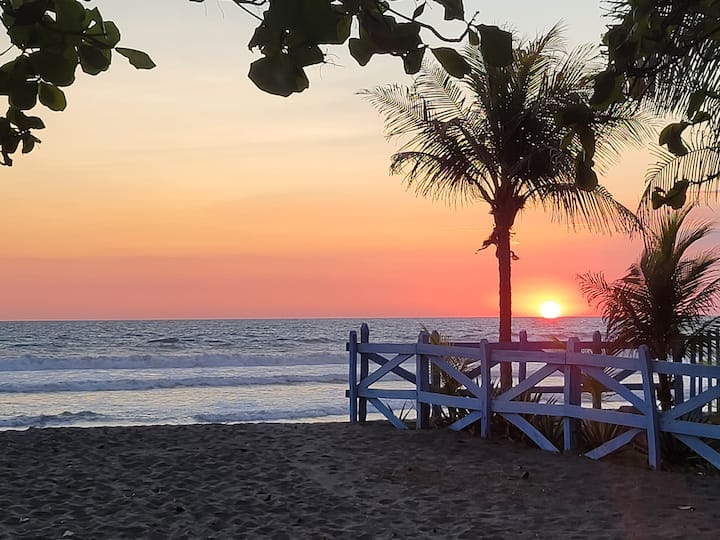This photograph captures a serene beach scene at sunset. In the foreground, there's a stretch of gray, sandy beach. On the right side, a blue and white wooden picket fence encircles an area with various trees and plants, including a noticeable palm tree near where the sun is setting. The light blue sea with gentle waves extends towards the horizon, where the vibrant sky showcases a gradient of colors—red at the bottom, transitioning to yellow, cream, and then blue as it ascends. The setting sun, appearing white, casts a yellow hue on the surrounding sky, adding to the ethereal quality of this picturesque moment.